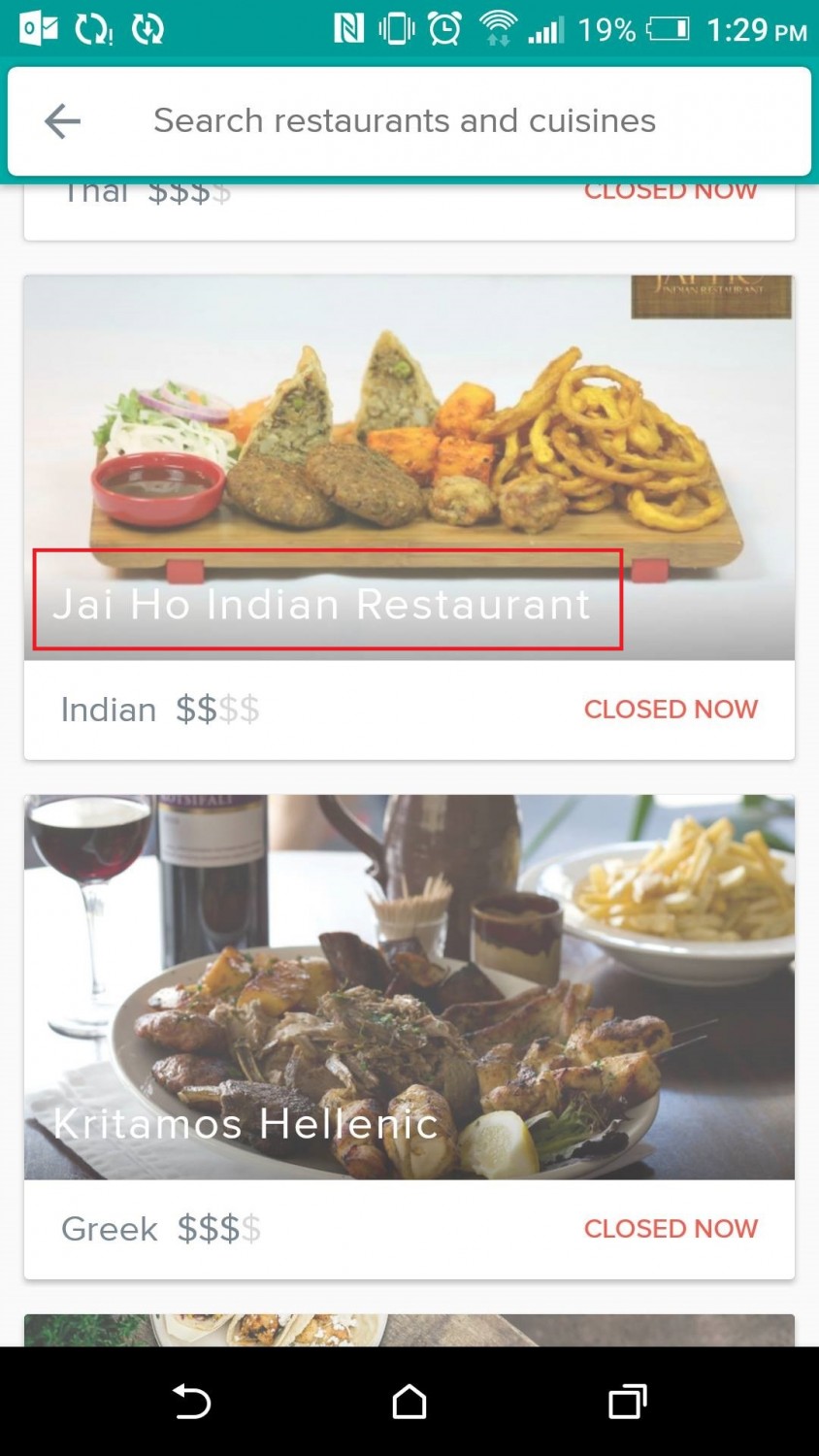**Category: Websites**

The image features a phone screen displaying a food delivery app interface. At the very top of the screen, the status bar shows several icons: an email notification, a refresh button, a vibrate mode indicator, an alarm symbol, Wi-Fi connectivity, a battery level at 19%, and the current time, 1:29 PM.

Below the status bar is a search bar with a white field bordered by teal, reading "Search restaurants and cuisines." It includes a back arrow for easy navigation. Partially visible below the search bar is a listing for a restaurant specializing in Thai cuisine, marked as currently closed and indicated by three dollar signs ($$$), though detailed information about this restaurant isn't fully shown.

Below the Thai restaurant listing, a highlighted entry is for "Jai Ho Indian Restaurant." The image accompanying this entry displays a variety of food on a wooden serving platter. The foods include what looks like onion rings, naan bread, a white sauce, some kind of patties, and an orange item, likely a root vegetable.

Further down the screen, there's another restaurant listing for "Kretamos Hellenic," denoted as Greek cuisine with three dollar signs ($$$). The image here depicts a dish of pasta, potatoes, grape leaves, a cup, and a glass of wine in the background, suggesting a traditional Greek meal setting.